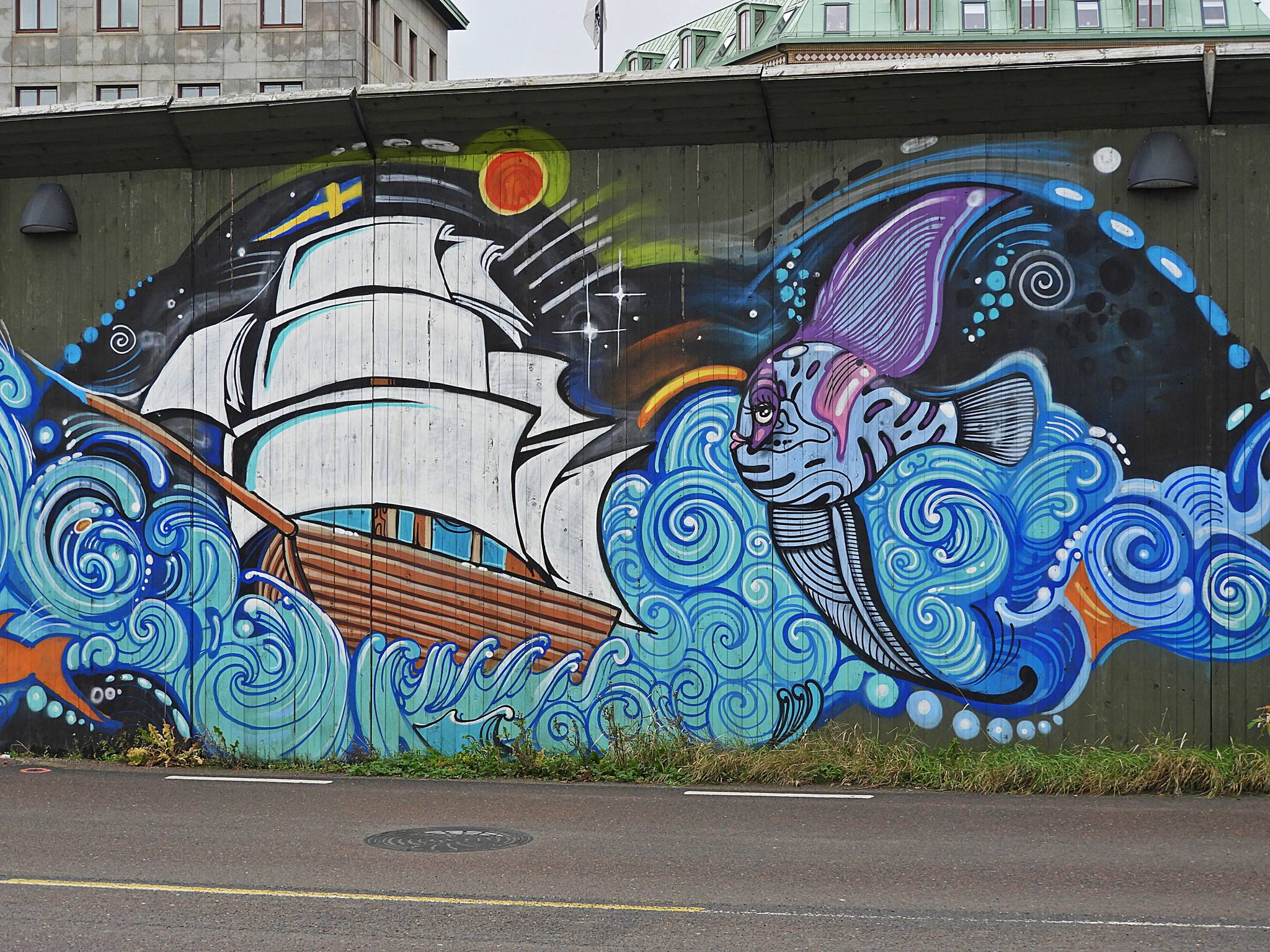This is a daytime outdoor photograph capturing a vibrant streetside mural painted on the vertical wooden slats of a building. The lower portion of the photograph shows a paved road with a manhole cover and a yellow center line, grounding the scene in an urban environment. Dominating the upper portion of the image, the mural features an antique sailing ship with white sails, a blue flag with a yellow cross, and a prominent figurehead jutting out from the bow, all floating on swirling blue waves. Above the ship, a striking red circle, possibly representing the sun or moon, and some constellations add celestial elements against a dark background. To the right of the ship, a large blue-purple angelfish swims leftward, blending into the watery hues. Peeking over the mural's building, stone structures are visible on both the left and right sides, adding depth to the scene. The mural is rich in color, primarily featuring shades of blue with touches of brown, red, and orange, depicting a fantastical maritime scene.